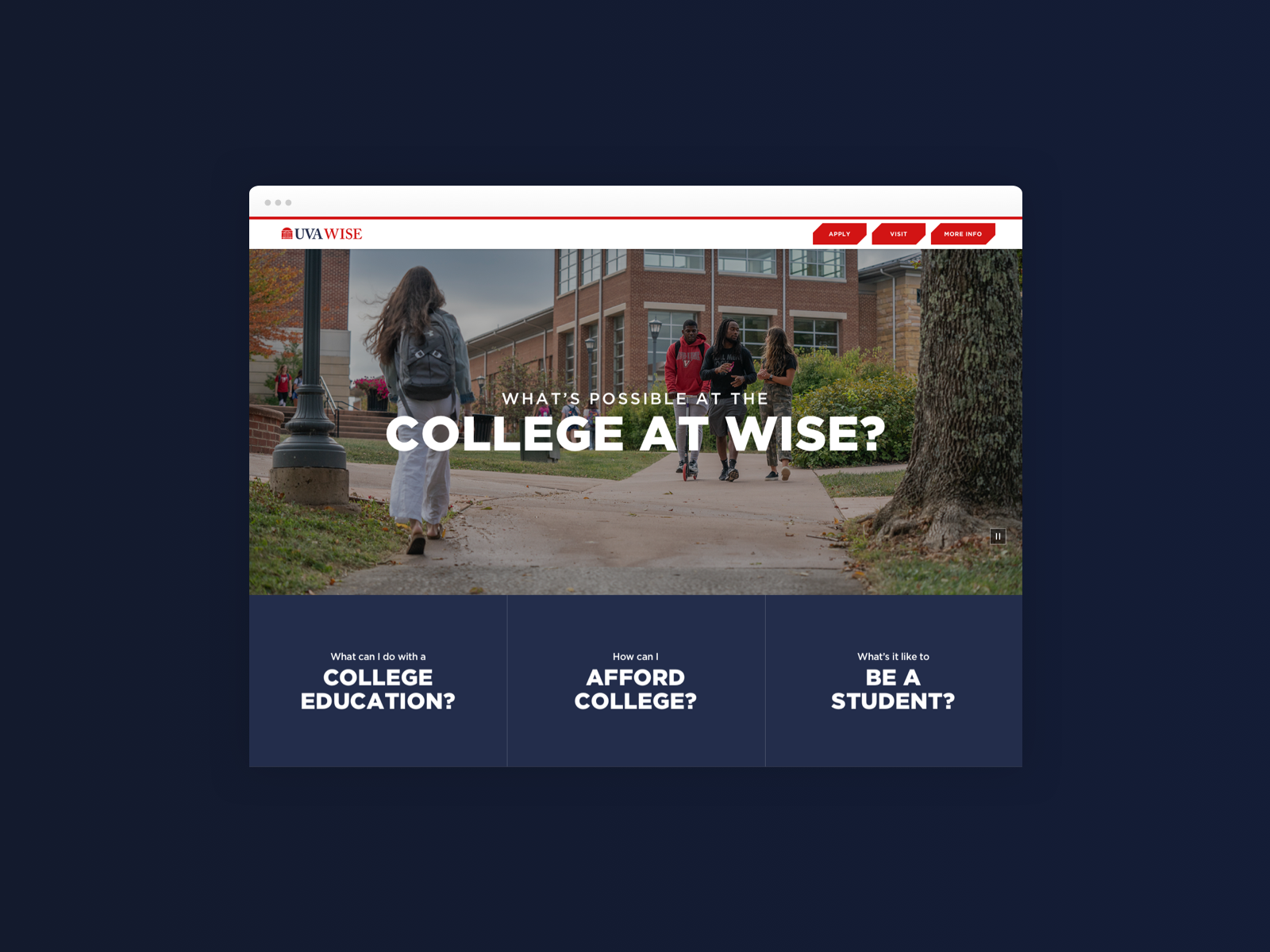This screenshot from a UVA WISE college advertisement features a predominantly dark blue background with a central pop-up. The pop-up presents a white header adorned with red text, which prominently displays "UVA" in black followed by "WISE" in red. On the right side of the pop-up are three red tabs labeled "Apply," "Visit," and "More Info." 

The image within the pop-up showcases a vibrant college scene. There’s a modern brick building in the background, exuding contemporary architectural elements. The foreground captures three students walking together in one direction, while another student heads in the opposite direction, exemplifying the daily hustle and bustle of college life. A lamp post can be seen on the left side of the scene, with a tree positioned to the right, adding a touch of nature to the campus pathway.

Text at the top of the image reads "What's Possible at the College at WISE," with "College at WISE" emphasized in large, uppercase font. At the bottom, a black header spans the width of the image, divided into three informative sections. The first section asks, "What can I do with a college education?" The middle section inquires, "How can I afford college?" And the final section poses, "What is it like to be a student?"

This detailed, visually engaging ad aims to provide prospective students with a glimpse into the vibrant and promising life at UVA WISE.